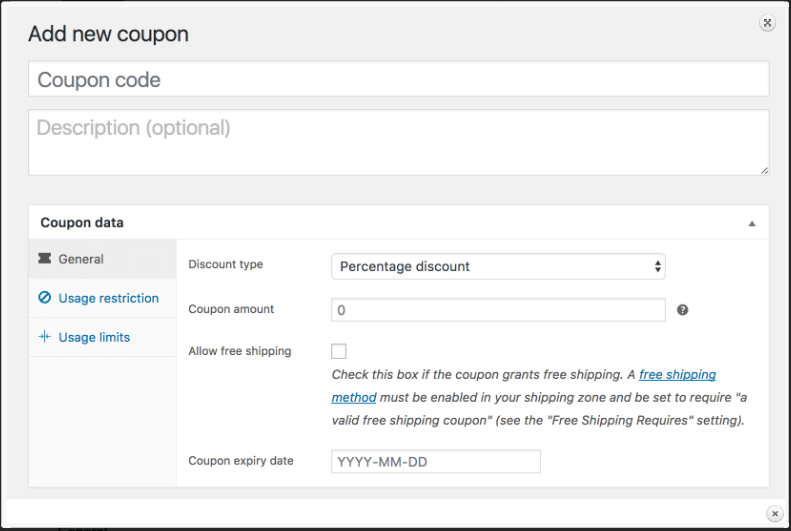**Screenshot Description: Adding a New Coupon on a Website**

The image is a screenshot from a website interface for adding new coupons. The section title "Add New Coupon" is prominently displayed at the top left corner. Below the title, there are two vertically stacked text fields. The first text field, positioned directly beneath the section title, includes a placeholder text that reads "Coupon Code." The second text field, located immediately below the first, has the placeholder text "Description (optional)," with the word "optional" indicated in brackets.

Further down, there is another section titled "Coupon Data." On the left side of this section, there are three buttons arranged vertically. The first button, labeled "General," is displayed in gray text, while the other two buttons labeled "Usage Restriction" and "Usage Limits" are in blue text.

On the right-hand side of the "Coupon Data" section are four distinct fields:

1. **Discount Type:** This field includes a placeholder text that states "Percentage Discount."
2. **Coupon Amount:** This text field has a placeholder text reading "0."
3. **Allow Free Shipping:** Next to this label is a checkbox accompanied by a line of explanatory text: "Check this box if the coupon grants free shipping. A free shipping method must be enabled in your shipping zone and be set to require a valid free shipping coupon. See the free shipping requires setting." This checkbox is currently unchecked.
4. **Coupon Expiry Date:** The final field has a placeholder text formatted as "YYYY-MM-DD."

The image captures a structured and user-friendly interface designed to facilitate the addition of new coupons efficiently.